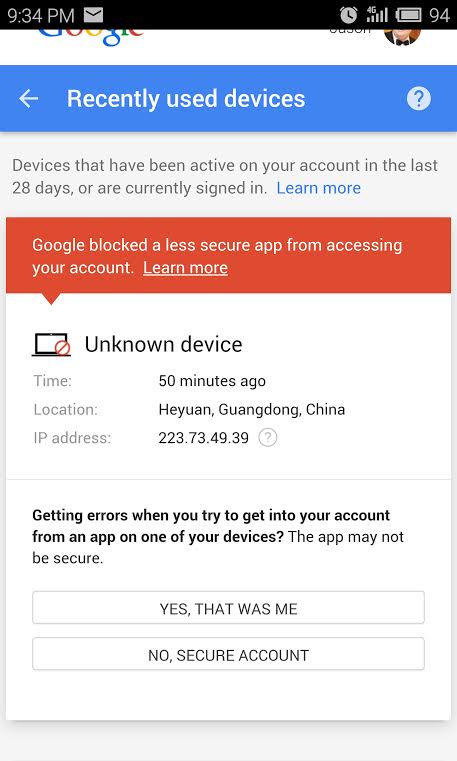This is a detailed screenshot of a smartphone taken from a website or alert notification. The screenshot reveals the time, which is 9:34 PM, visible in the top left corner, and the battery charge level, showing 94%, located in the top right corner. Also visible in the top left is a partial view of the Google logo, along with the bottom half of the user's profile picture at the top right.

The header of the screenshot displays the text "Recently used devices" against a blue background banner. Just below this header, there's a statement explaining that the section lists "devices that have been active on your account in the last 28 days or are currently signed in," along with a clickable "Learn more" link in blue.

Beneath this information, an orange alert box prominently states, "Google blocked a less secure app from accessing your account," accompanied by an underlined "Learn more" link for additional details. Following this alert, the notification specifies the device in question as an "Unknown device," highlighting that the attempted access occurred 50 minutes ago from the location "Heyuan, China." This indicates an unauthorized login attempt from a foreign country, which was successfully blocked by Google's security measures.